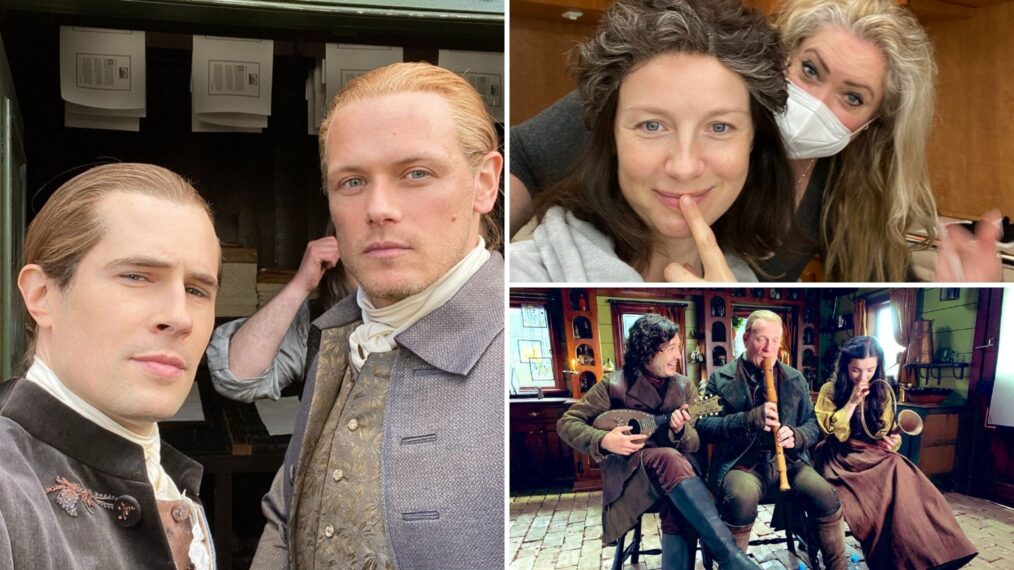The image is a color collage composed of three photographs featuring people dressed in historical or period attire. On the left, a large vertical photograph shows two men in dark Renaissance or Victorian clothing, complete with suit coats, vests, and scarves tied around their necks; both men have their hair pulled back into ponytails. In the upper right corner, a horizontal photograph depicts two women: the woman in the foreground, with black and gray hair, is holding a finger to her lips in a shushing gesture, while the woman behind her, peeking out with long blonde hair and wearing a surgical mask, looks directly at the camera. The lower right corner contains another horizontal photograph of three individuals playing musical instruments typically seen at Renaissance fairs. One person, dressed in brown attire and black boots with long, curly white hair, is playing a mandolin. Beside him, another man is playing a flute, and a woman with long brown curly hair is playing a horn. They are positioned in what appears to be a home setting, sitting on stools. All the photographs share a cohesive theme of historical reenactment or costume, suggesting scenes one might encounter at a Renaissance fair.